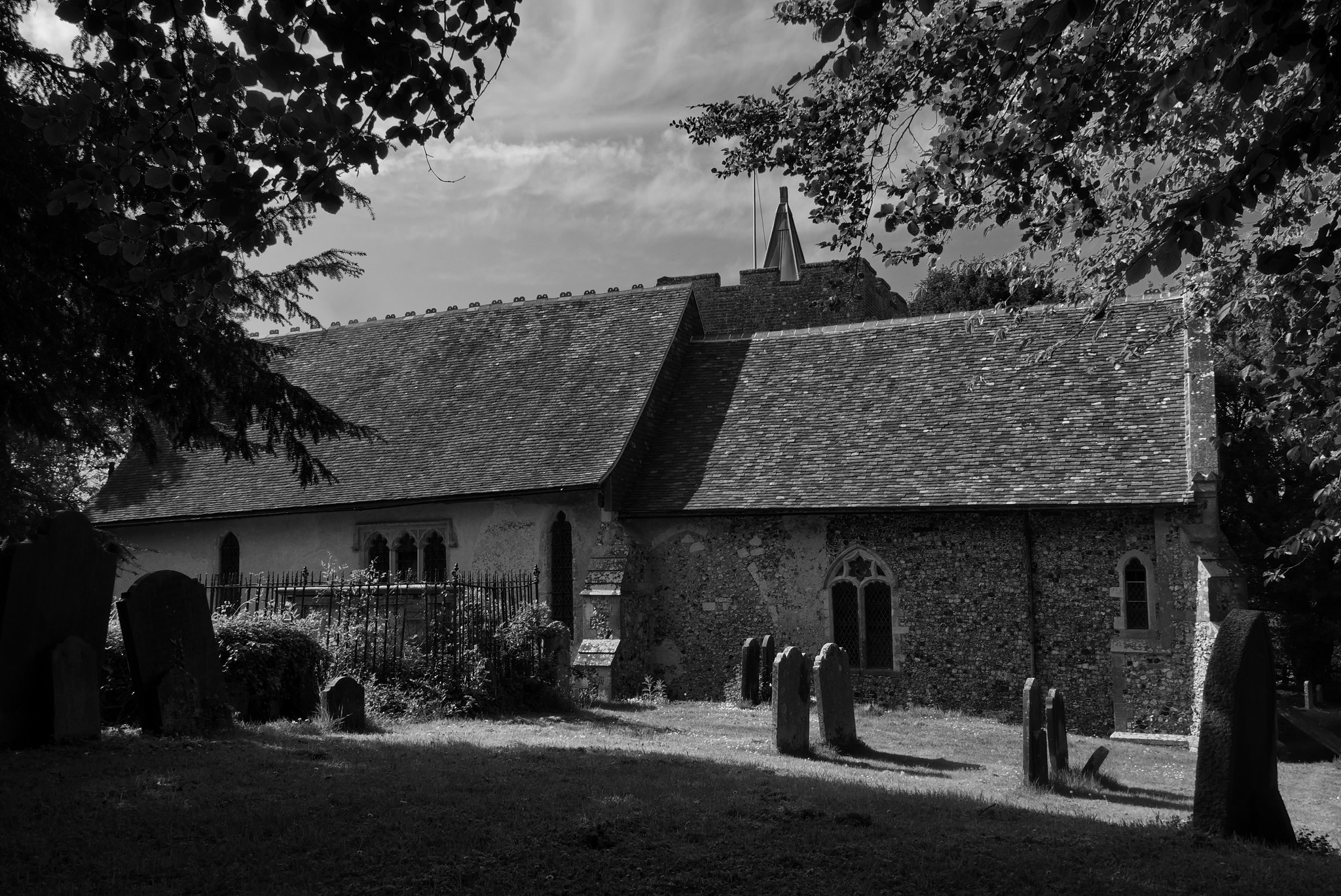A historical black and white photograph showcases an old church building, likely dating back to the early 1900s. The structure is primarily constructed of brick, contrasted by a dark-colored roof. A prominent steeple crowns part of the building, while arched windows of varying sizes punctuate the walls—one smaller window on the side and a larger, more imposing one nearby. 

In the foreground, a charming black iron fence encloses the church's cemetery, where several gravestones, approximately eight to ten, are visible. The cemetery is dotted with bushes and dominated by a towering tree, adding to the serene atmosphere. A little sign leans against the side of the church, which reveals more windows and an interesting architectural detail: the front half of the building appears to be made of concrete rather than brick. Overall, the picturesque church, with its rich history and quaint details, exudes a timeless beauty.